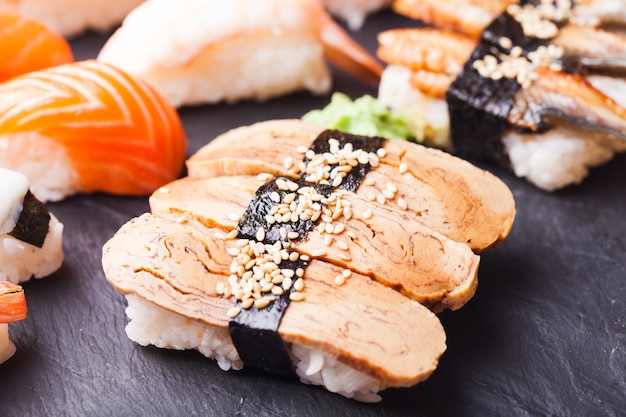A detailed close-up photo of a sushi plate, prominently featuring three pieces of tamago nigiri. Each piece consists of a mound of white rice topped with a flat, beige slice of Japanese egg omelet, all wrapped together with a strip of seaweed and sprinkled with sesame seeds. The sushi sits on a black, textured surface resembling natural stone. Behind the tamago nigiri, slightly out of focus, are various other sushi pieces including a raw salmon nigiri with pink salmon over white rice, and grilled fish nigiri types such as shrimp and eel, some of which are also wrapped in seaweed and garnished with sesame seeds.